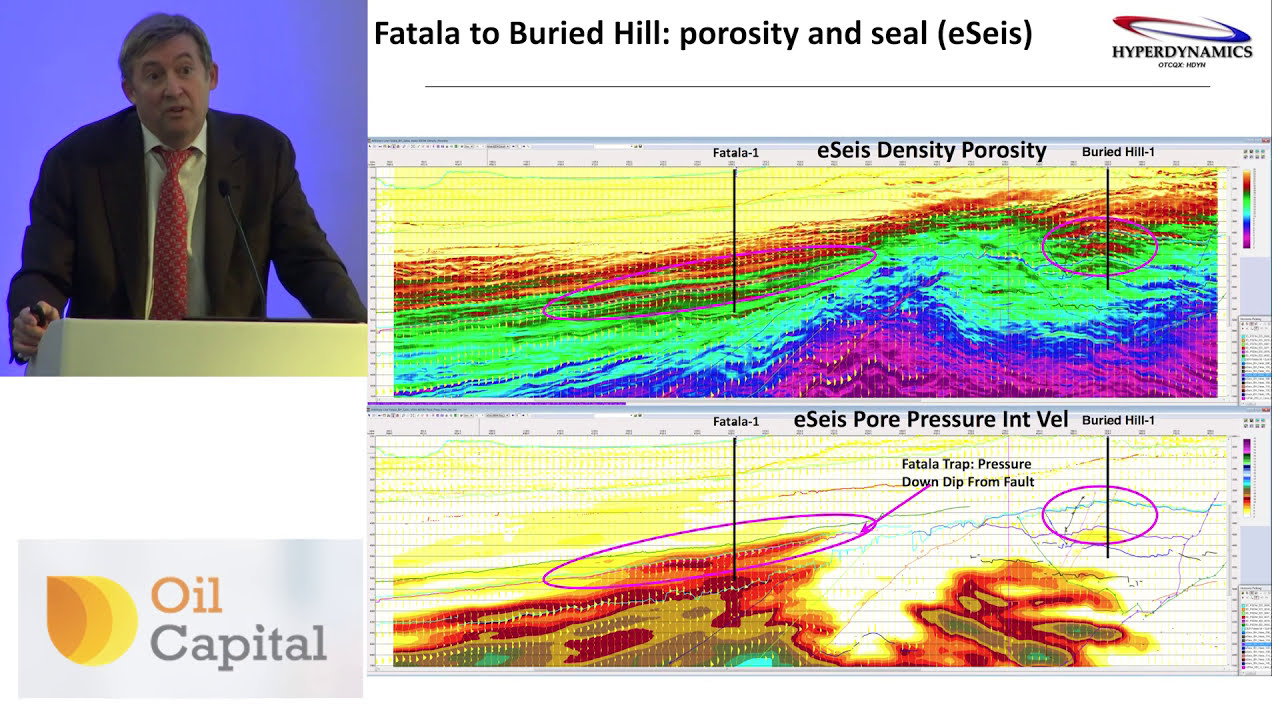The image captures a detailed scientific presentation focused on hyperdynamics and oil exploration. Dominating the upper-left corner is a video window featuring a man at a white podium with a microphone. He has short gray hair and wears an open black suit coat, a red tie with a thin white stripe diamond pattern, and a white button-up shirt. The slide prominently reads "Fatala to Buried Hill Porosity and Seal" with the acronym "E.S.E.I.S" next to it, indicating a technical aspect of the presentation. The top-right corner showcases intertwined red and blue half circles labeled "hyperdynamics." Below, two colorful thermographs display data on ESIS density and porosity, using vivid hues like purple, blue, green, yellow, red, and violet. These thermographs are annotated with terms such as "Fatala Trap Pressure Down Dip from Fault" and "Buried Hill," suggesting geological characteristics and the locations of oil reserves. At the bottom of the slide, the term "Oil Capital" signifies the economic focus of the presentation, further emphasized by discussions on oil pressure and optimal extraction sites.